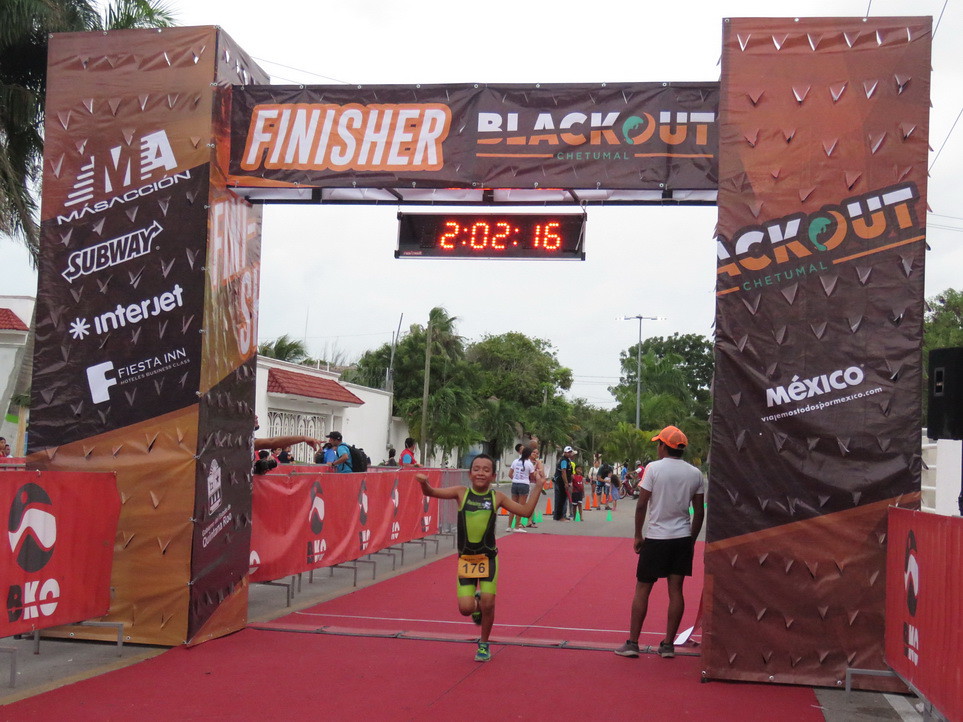In this image capturing the dramatic end of a marathon, a young boy with tan skin and black hair bursts through the finish line with his arms triumphantly raised. He is clad in a green and black spandex suit, prominently displaying the number 176. The finish line itself is framed by an archway constructed from vinyl banners stretched over a wire structure, adorned with various sponsor logos such as Subway, Interjet, and Fiesta Inn, all set against a predominantly brown backdrop. Dominating the archway is a sign reading "Finisher" in bold white letters within an orange box, alongside the logo for "Blackout Chantunel," featuring unique brown and white text with a swirling 'O' encasing a green fish. Below this, a digital display marks the finishing time: 2 hours, 2 minutes, and 16 seconds. The scene is set on a red-carpeted track area, bordered with gray and red barriers, adding a touch of grandeur to the event. In the background, several spectators line up to witness the event, amidst tall palm trees and under slightly overcast skies, suggesting a tropical locale, possibly Chetumal, Mexico. Additionally, another individual stands at the finish line, overseeing the proceedings, dressed in a white t-shirt, black shorts, and an orange-billed cap. The overall environment hints at a festive yet modestly attended event, complete with stadium lights in the distance.